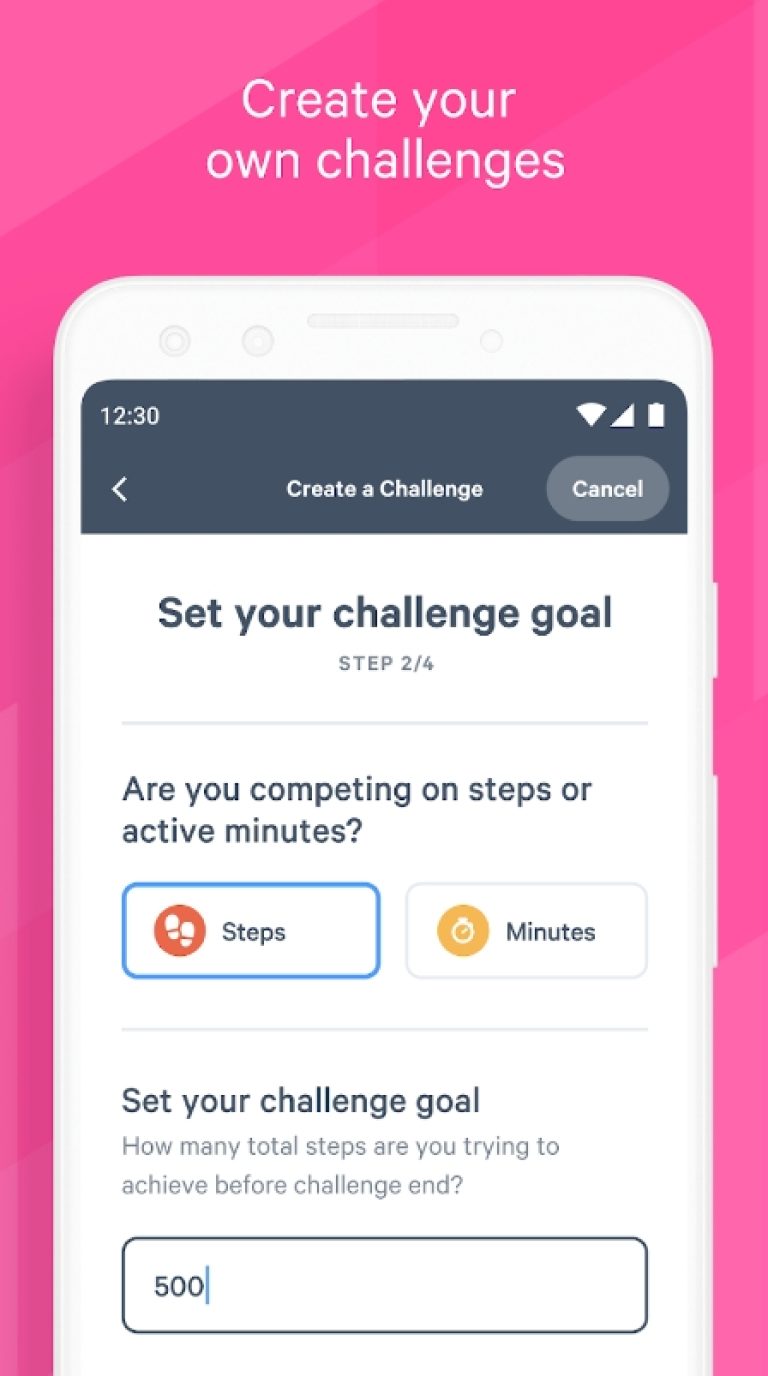The image features a design for a cell phone screen with a distinct border and detailed user interface elements. The outer border is pink, encompassing the left, right, and top edges of the screen. At the very top of the image, there's white text on the pink background that reads "Create Your Own Challenges."

The cell phone screen itself has a mostly white background. The very top of the screen is black, displaying standard phone status indicators including "12:30," a Wi-Fi connection icon, and a battery icon. Immediately below these indicators is the title "Create a Challenge," with a gray "Cancel" button to its right.

The middle portion of the screen features the instruction "Set your challenge goal, step 2 of 4" in black text. Below this, there's a question asking, "Are you competing on steps or active minutes?" There are two options to respond: the first option, outlined in a blue rectangular border, is labeled "Steps," and the second option is labeled "Minutes."

Toward the bottom of the screen, another instructional prompt reads, "Set your challenge goal: How many total steps are you trying to achieve before the challenge ends?" Immediately below this prompt, the number "500" is typed out in a text field, indicating the goal for total steps. This completes the design elements presented in the image.